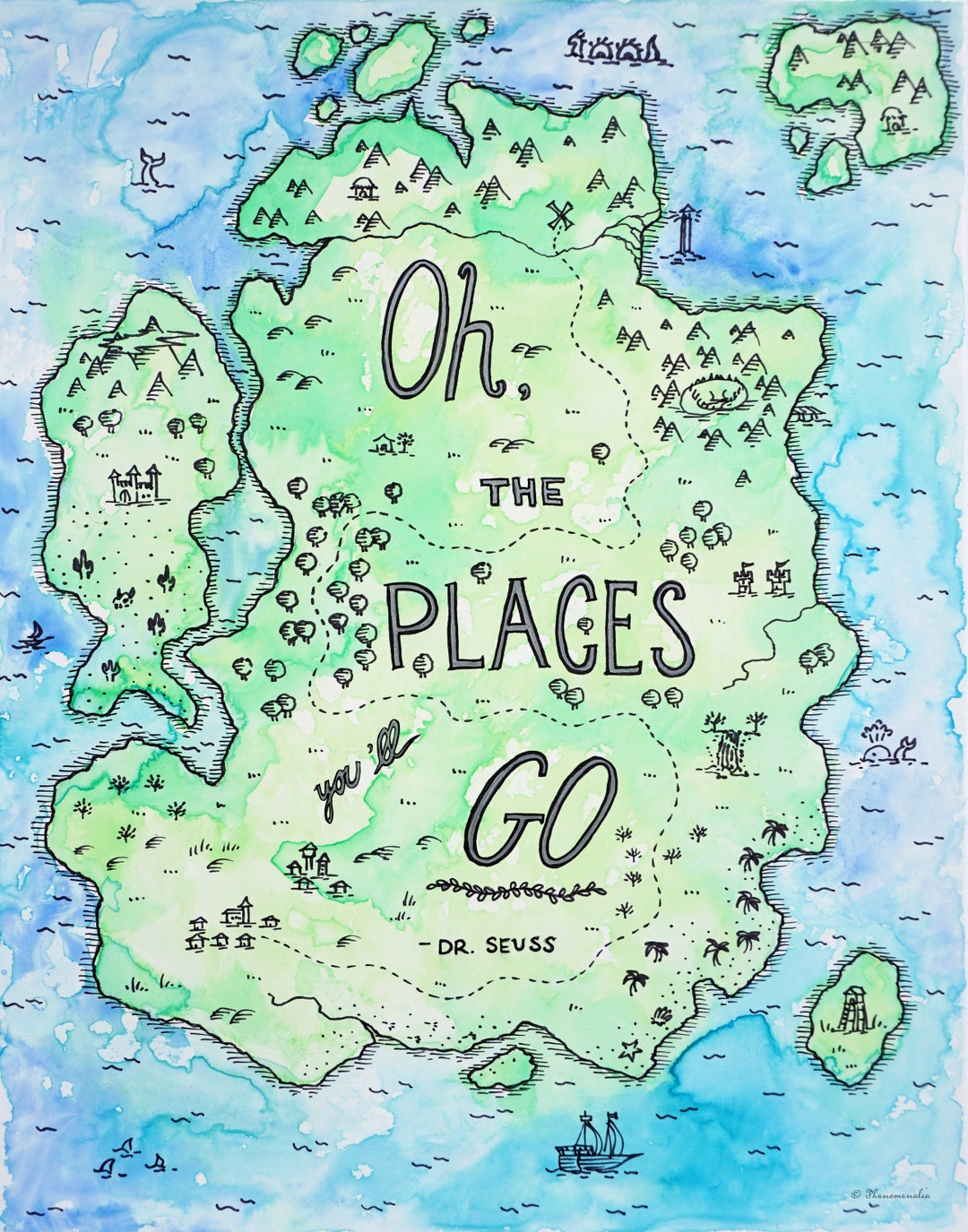This is an intricately illustrated, multi-color map that is vertically rectangular with no distinctive border or specific background. The centerpiece of the map is a large island surrounded by multiple smaller islands. The main island features text prominently arranged as follows: at the top in ornate cursive it reads, "O, THE PLACES YOU’LL", and at the bottom in larger print, "GO", with the signature "Dr. Seuss" beneath it.

The artwork is drawn in a style reminiscent of colored pencil, with vibrant hues bringing life to the depiction. The central island is detailed with trees and mountains, hinting at various adventures. Surrounding the primary island are several smaller ones, each unique; one has a castle, another a lookout or lighthouse, and a cluster of five smaller islands sits above to the left.

The water, rendered in shades of light and dark blue, is filled with engaging illustrations of sea creatures and vessels. Sketched whimsically in the waves are birds, a sailboat, people in a canoe, a dragon, a whale's tail, and a Loch Ness monster-like figure. Additionally, the map shows a dotted path, suggesting an adventurous route to be taken across the islands and waters. Subtle details such as black specks and faint outlines add to the mystique of the scene, making this map not just a guide, but an invitation to explore the imaginative world of Dr. Seuss.